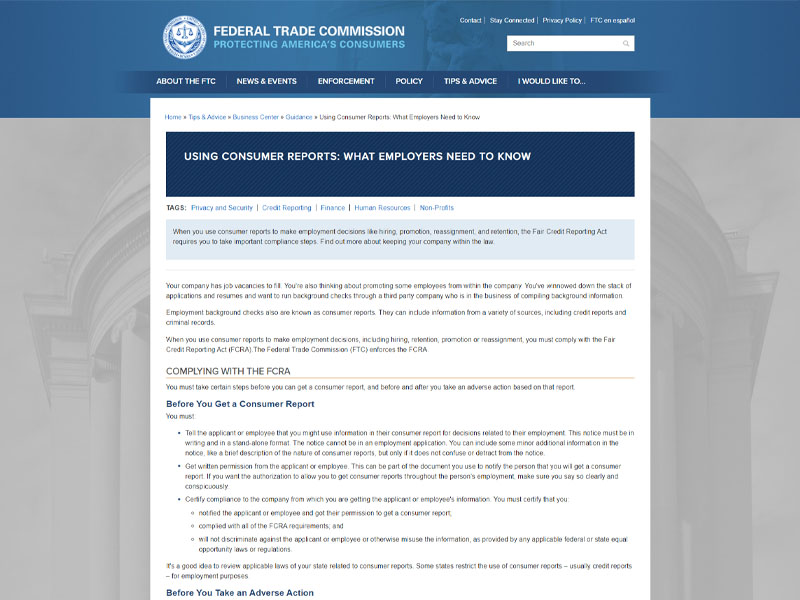The webpage from the Federal Trade Commission (FTC) features a prominently blue-themed header. On the top left, the FTC logo is displayed, followed by the text "FEDERAL TRADE COMMISSION" in bold, white, all-capital letters. Beneath this, in a slightly smaller, light-blue font, is the motto "PROTECTING AMERICA'S CONSUMERS."

To the upper right of the header, there are several horizontally aligned links: "Contact," "Stay Connected," "Privacy Policy," and "FTC en Español." A white search box is situated directly below these links, providing visitors with a convenient search function.

Just below the header is a navigation bar with a darker blue background, featuring all-capital white text. The navigational buttons read: "ABOUT THE FTC," "NEWS AND EVENTS," "ENFORCEMENT," "POLICY," "TIPS AND ADVICE," and "I WOULD LIKE TO."

In the main content area of the page, a document titled "Using Consumer Reports: What Employers Need to Know" is prominently displayed, offering essential guidance for employers regarding the use of consumer reports.